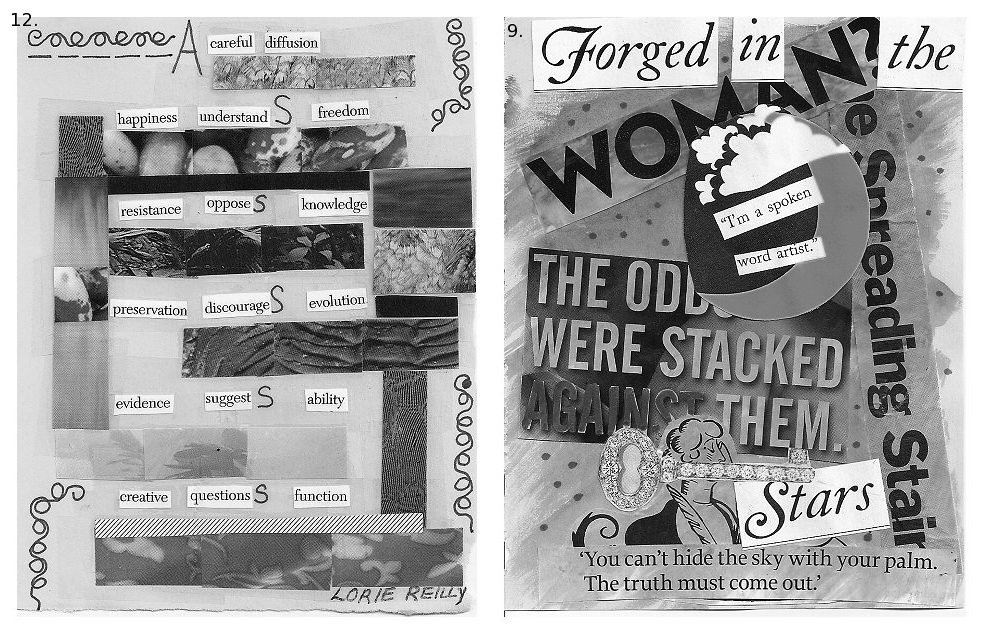The image displays two intricately designed scrapbook-style pages, each with a distinct set of elements and a grayscale aesthetic. The left page features the number "12." at the top, followed by a collage of carefully cut-out words and phrases from magazines, interspersed with handwritten elements. The collage reads: "a careful diffusion happiness understands freedom resistance opposes knowledge preservation discourages evolution evidence suggests ability creative questions function." Various snippets of pictures and a signature by Lori Riley embellish this page, adding to its structured yet eclectic appearance.

The right page, marked with the number "9." at the top, continues this artistic style with more magazine cutouts and phrases. Prominent words and phrases include: "Forged in the", "woman?", "I'm a spoken word artist", "the odds were stacked against them", and "stars". It also features an image of a person from the 1920s with an illustration of a key over it, and a cut-out moon with clouds nearby. At the bottom, a poignant quote reads, "You can't hide the sky with your palm. The truth must come out.", alongside a strip with wording partially legible as "the spreading stare" or "stain". Symbols of resistance, creativity, and the pursuit of knowledge are embedded throughout this page, creating a narrative of resilience and expression.